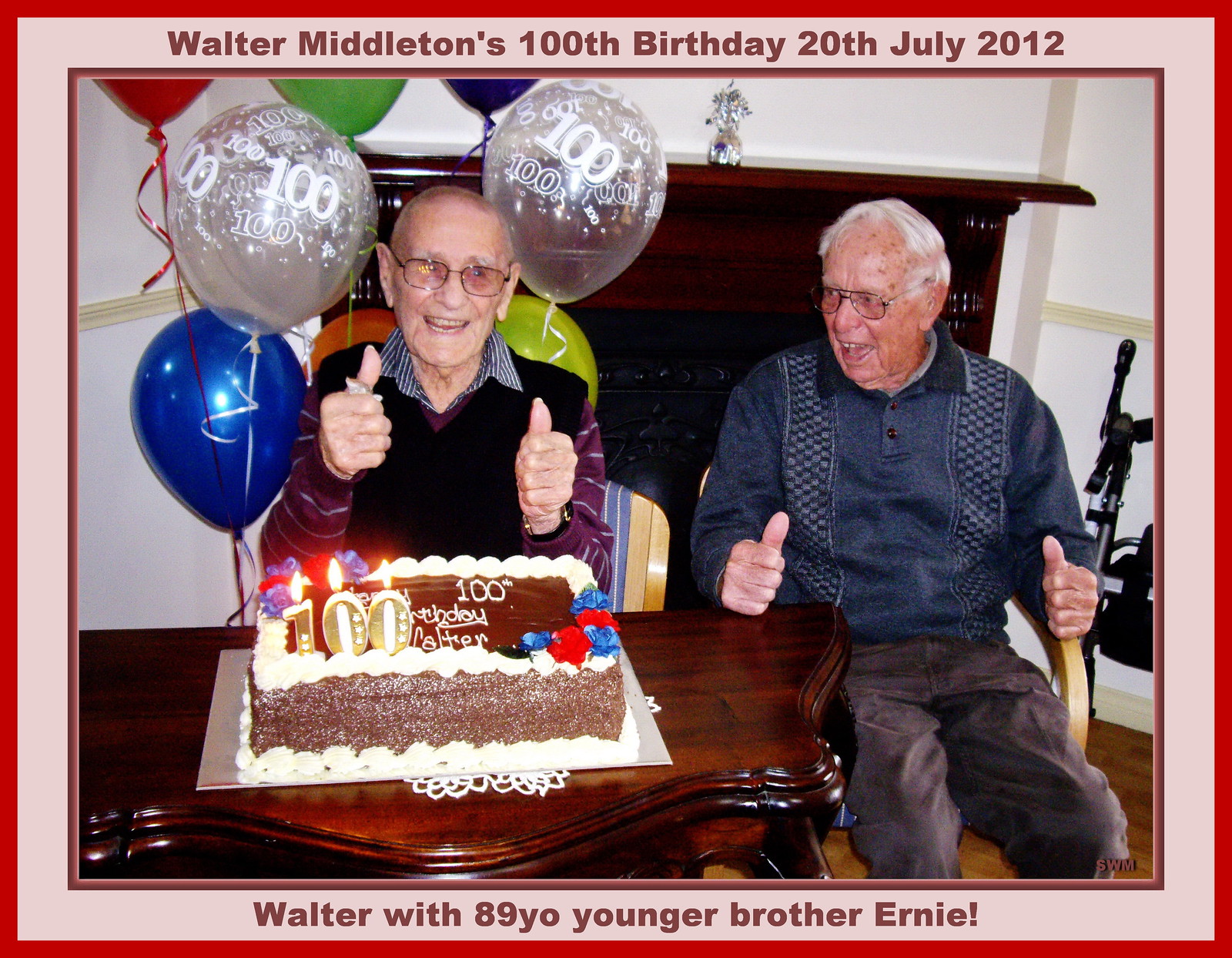The photograph captures a celebratory moment featuring two elderly men, Walter Middleton and his younger brother Ernie, in a white room. The image, framed by a pink and red border, is marked with text at the top that reads "Walter Middleton's 100th birthday, 20th July 2012," and at the bottom it states, "Walter with 89 year old younger brother Ernie."

Walter, at the center of the photograph, sits in a brown armchair with his thumbs up, wearing a striped maroon shirt, a black vest, and dark slacks. He is smiling directly at the camera. Beside him, Ernie, who has white hair, glasses, and liver spots, is looking affectionately at Walter, also giving a thumbs-up. Ernie is dressed in a gray sweater and slacks, spotted behind him is a walking cane. Both men exude joy in their expressions.

In front of Walter is a dark cherry wood table adorned with a doily and a celebratory chocolate cake decorated with red and blue icing and topped with candles spelling out "100." The atmosphere is festive, further highlighted by an array of colorful balloons in blue, red, purple, green, clear, white, yellow, and orange. The room also features a matching cherry wood fireplace behind the brothers and a polished hardwood floor, adding warmth to the scene.